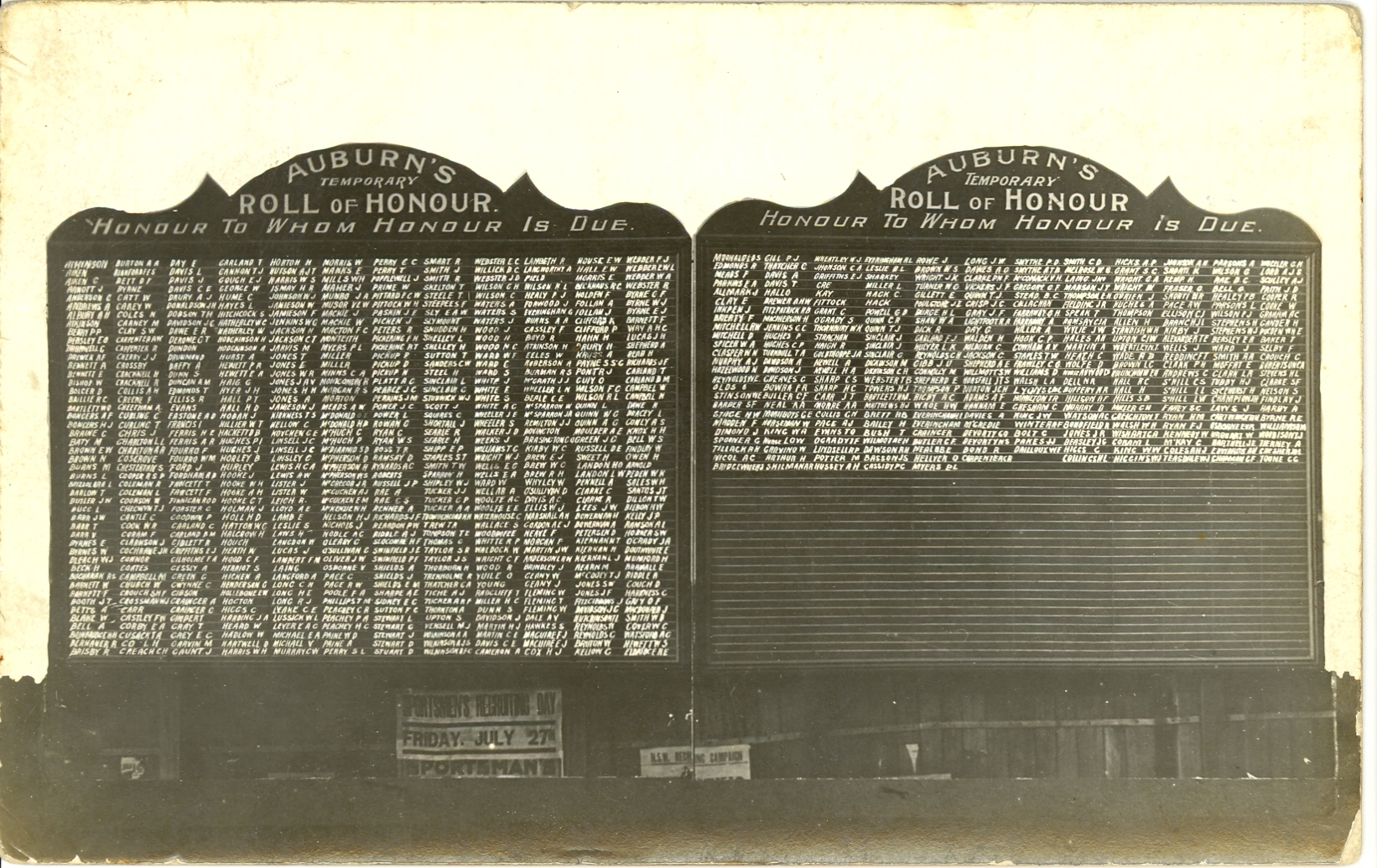The photograph, a yellowed and weathered rectangular image, showcases two adjacent black plaques with a shared curved top design featuring triangular points on either side. Both plaques prominently display the title "Auburn's Roll of Honor" followed by the phrase "Honor to whom honor is due." Each plaque contains 12 columns inscribed with numerous names in white text. The first plaque is fully filled with names, while the second plaque is only half-filled. Below these plaques is a black banner announcing "Sportsman's Recognition Day, Friday, July 27th." The age of the photo is apparent, with visible creases and browning at the edges.